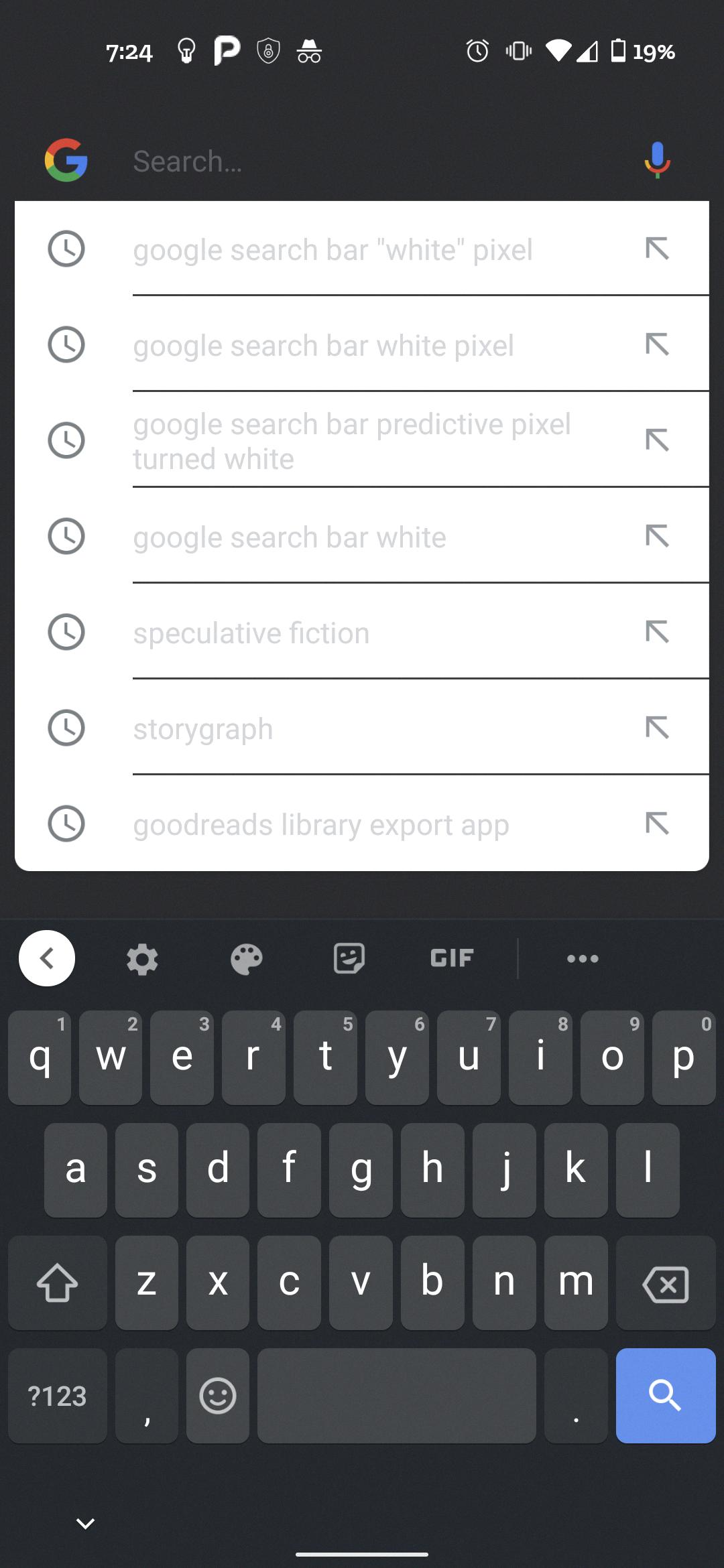This is a highly detailed visual description of a smartphone screenshot:

The screenshot captures the smartphone screen in a vertical orientation, with a black background. At the top-left corner of the screen, the time is displayed as 7:24 AM. Adjacent to the time are several icons: a light bulb, a "P," a shield, and a hat with round glasses underneath. 

On the top-right corner, additional icons are visible, including an alarm clock, a vibrate icon, Wi-Fi signal bars, cellular signal strength, and a battery icon indicating a 19% charge remaining. 

Just below this row of icons is the Google search bar. This bar features the Google "G" logo on the left side and a microphone icon on the right side. 

Beneath the search bar is a white rectangular area featuring seven lines of text, each separated by a thin gray horizontal line. The texts are as follows:
1. "Google search bar white pixel"
2. "Google search bar white pixel"
3. "Google search bar predictive pixel turned white"
4. "Google search bar white"
5. "Speculative fiction story graph"
6. "Goodreads library export app"

Each line of text has an arrow icon on the right, which points diagonally towards the upper left, indicating the presence of additional information or a link associated with each entry.